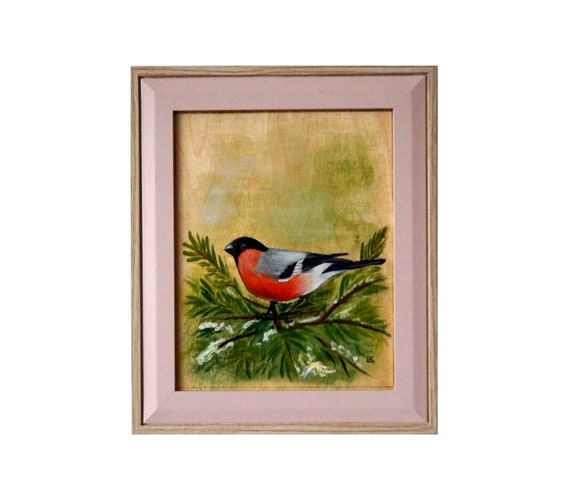Framed within a thin, light-colored pink wooden frame is a vertical painting set against a beige and gold-green patchy background, evocative of wood grain. This painting depicts a small, vividly colored bird perched on what seems to be a conifer branch. The bird, the main subject of the painting, has a small black head, a tiny black beak with a grayish reflection, red plumage covering its chest and belly, and a mix of gray and black on its wings. Its tail feathers are white tipped with black. The bird rests on branches adorned with sparse, needle-like green leaves and patches of snow, adding a sense of a wintry scene. The upper half of the painting features the blurred green and grayish shades, suggesting foliage or sky, rendered in a watercolor-like technique, leaving the bird and branches as the focal point in the lower half. The artistry of the piece, combined with the unique wood-textured backdrop and the detailed bird, creates a serene and natural winter tableau.